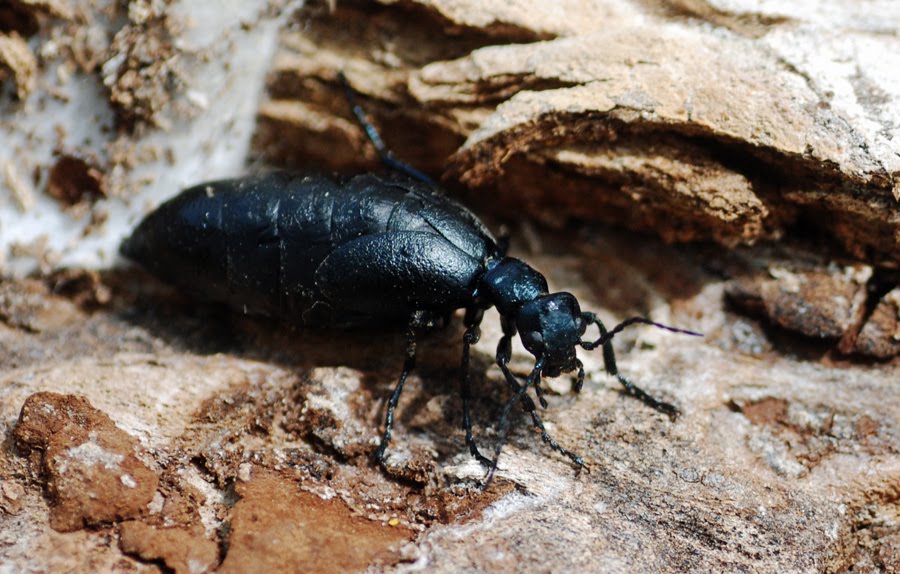The color photograph captures a black beetle on a rocky, sandy surface, featuring various shades of brown and cream. The landscape-oriented image highlights the beetle at the center, situated on top of reddish-brown shale rocks with a roughly textured, light-brown background. The beetle's head is slightly down, and its long, segmented antennae stretch out, almost touching the ground and pointing in opposite directions. The front legs are visible, segmented, and pointing toward the bottom right, though the rear legs are obscured by shadows. The beetle's body is notable for its large, elliptical, and fat black abdomen, which features a slightly raised ribbed effect with horizontal bands. The narrow throat behind the head gives it an ant-like appearance, which may suggest a species variation. The photograph uses a close-up perspective to emphasize the detailed texture and form of both the beetle and the rocky terrain.